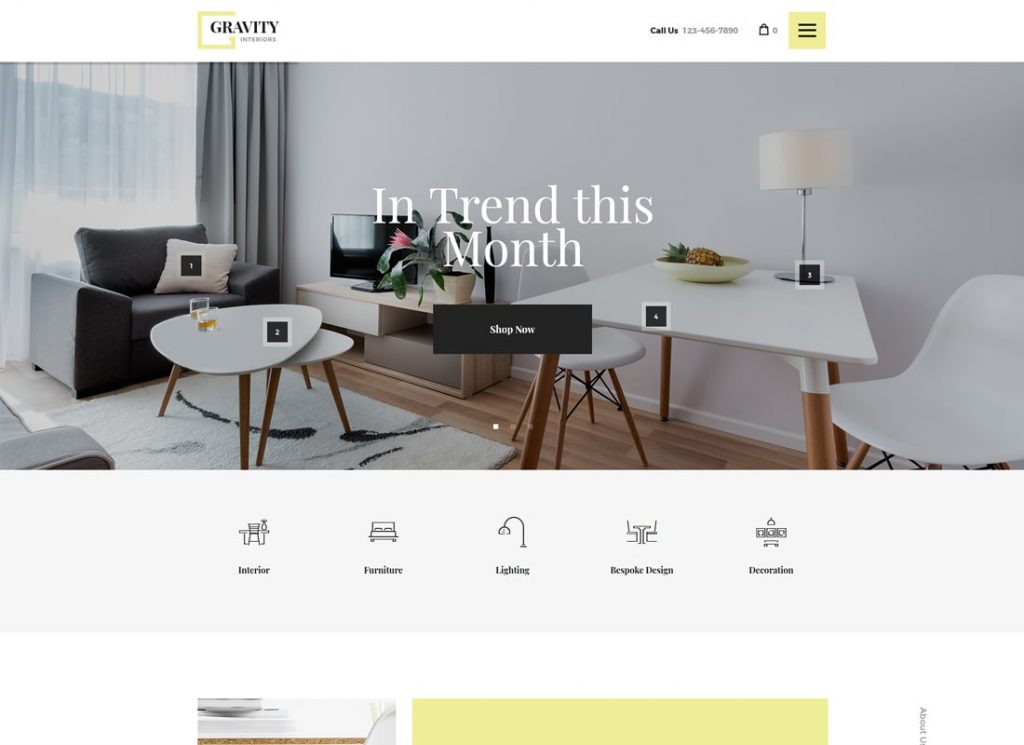A stylish interior designed by Gravity Interiors showcases this month's modern home trends. The room features an elegant combination of light grays and whites with contemporary furniture to create a sophisticated ambiance. Key elements include a sleek black single-seater sofa set in the corner, a compact TV stand, and lush houseplants adding a touch of green. The centerpiece is a chic table setup with stools, a modern lamp, and a decorative bowl holding a faux pineapple. Nearby, a small coffee table holds two glasses partially filled with what appears to be whiskey or brandy, enhancing the room's refined look. The carefully curated décor, including bespoke furniture and lighting, reflects a commitment to high-quality design. A 'Shop Now' button in black invites viewers to explore more, though a placeholder phone number indicates the website is still under construction.